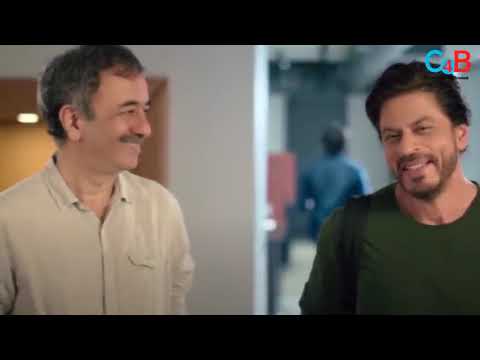In this blurry, pixelated still frame from a low-resolution movie or TV show, two men stand facing each other in what appears to be an office setting. The man on the right, who has dark brown hair and a light beard and mustache, is smiling warmly with his head slightly tipped to the right, revealing his top row of teeth. He is wearing a green sweater with a bag slung over his right shoulder. On the left is an older man, possibly in his late 40s or early 50s, with a mustache and salt-and-pepper hair around his ears. He is dressed in a tan button-down shirt with a front pocket and is gazing towards the man in the green sweater with a pleasant expression. Above them, there is a turquoise and red logo that seems to read "CAB" or "C4B," possibly indicating the network. In the background, another person in a blue shirt is seen walking in the opposite direction, further inside what seems to be an office, complete with partitions and an open doorway.